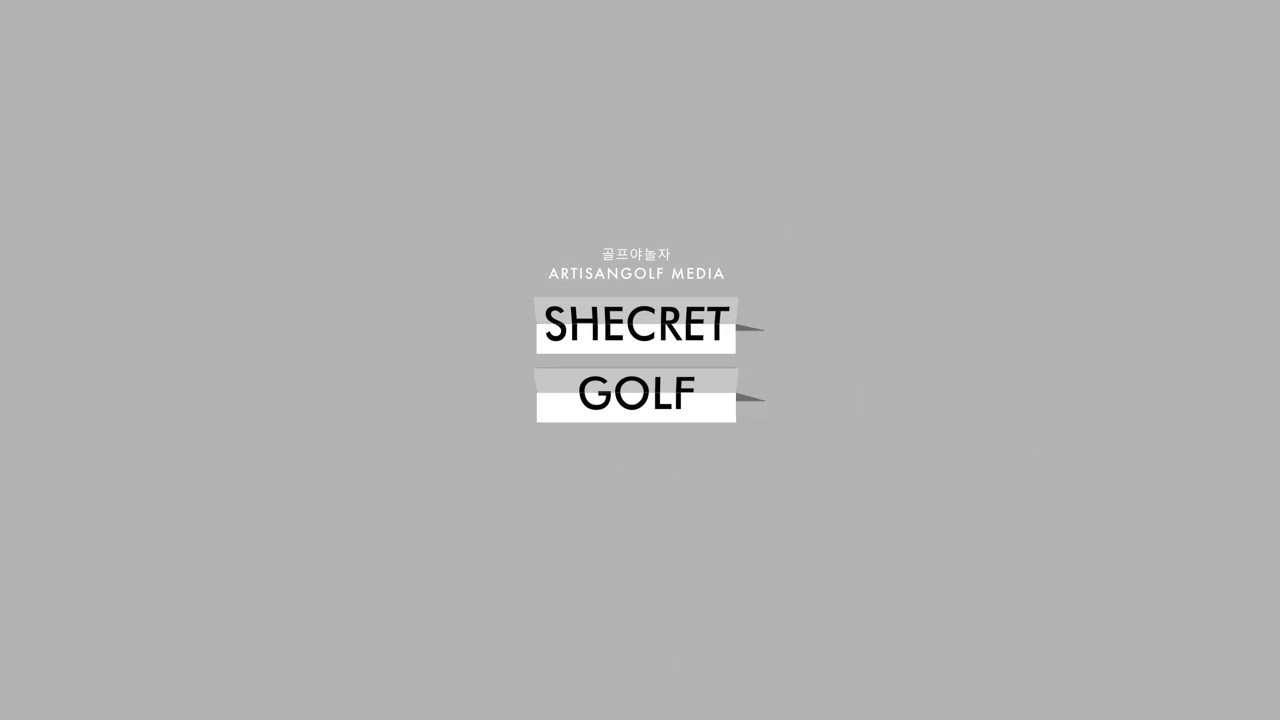This photograph captures an indoor yoga studio scene with a serene atmosphere, filled with various elements and textures. The studio's floor is made of light beige wooden planks, complementing the beige and brown tones of the walls, which feature stone tiles. The ceiling is adorned with fluorescent lighting, and natural light beams through the arches, adding a soft ambiance to the room. In the foreground, three young women, possibly teenagers, sit cross-legged on dark gray yoga mats positioned equidistantly across the floor. The central figure, wearing a navy blue spaghetti strap tank top and light blue yoga pants, rests her hands on her knees in a meditative pose. The woman on the left sports a salmon pink long-sleeve zip-up with black leggings, while the woman on the right is dressed in a navy sleeveless top paired with black leggings. Scattered around are exercise balls, brightening the space with their vibrant blue and lime green hues. In the background, a few more individuals can be seen, reinforcing the studio's purpose as a communal exercise space, ideally a yoga class in session.